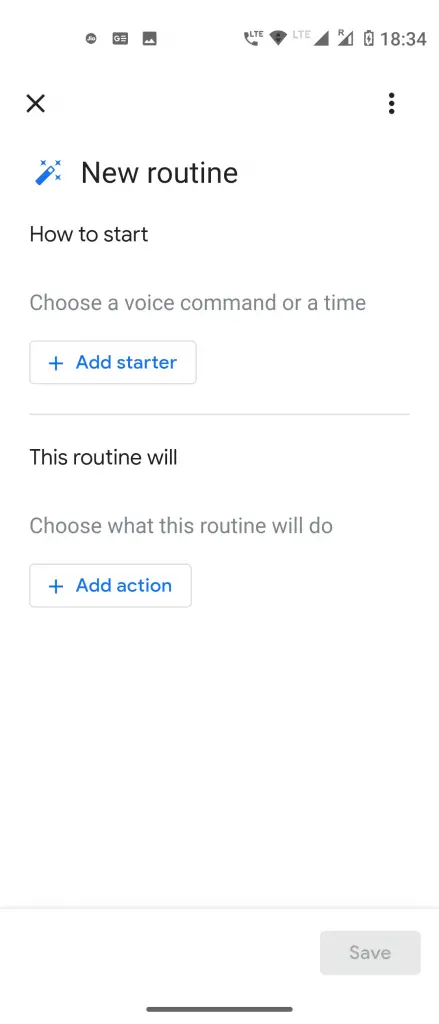The image is a screenshot of a mobile phone displaying a website interface focused on creating a new routine. At the top of the screen, the phone's status bar is visible, showing typical mobile phone indicators such as battery level, current time (18:34 or 6:34 PM), and internet connection status. 

In the upper-left corner of the interface, there is a prominent "X" button, likely for closing the current screen or dialog. To the right of the "X," three vertical dots suggest an additional options menu. Also on the top-left side, there is an icon resembling a wand with three sparkles, possibly indicating some sort of automation or magic feature.

The main content area begins with the heading "New Routine," which is bolded. Below this heading, the text "How to start" appears, followed by a prompt to "Choose a voice command or time." There is an actionable button labeled "Add Starter," marked with a plus sign.

Further down, the text "This routine will" introduces a section where users can specify actions the routine should perform. The prompt "Choose what this routine will do" is followed by another actionable option to "Add Action."

Overall, the interface looks user-friendly and easy to read, aimed at guiding users through the process of setting up a new routine with clear, step-by-step instructions.